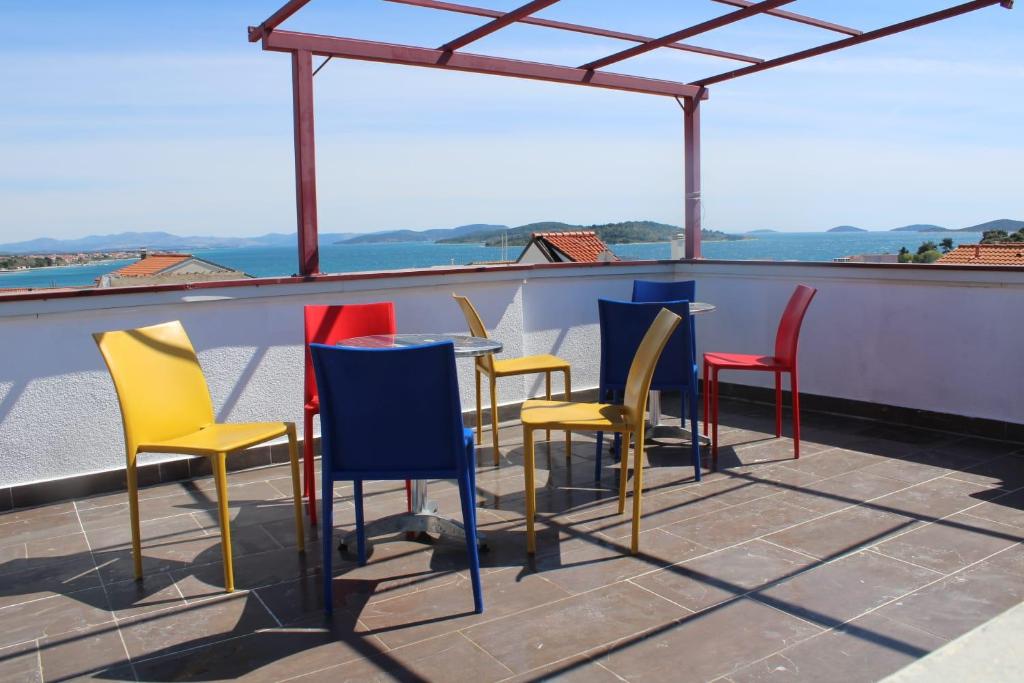The image shows a sunny outdoor deck that might be situated on a boat or a high patio area, surrounded by a white wall. The floor is covered with large gray tiles. It features two small round tables, each accompanied by simple, solid-colored chairs—yellow, blue, and red. The table on the left is surrounded by two yellow chairs, one blue chair, and one red chair, while the table on the right has two blue chairs, one yellow chair, and one red chair. The deck is open and exposed to the light, with a metal frame above that forms a checkered pattern but lacks a cover. In the background, you can see an expansive body of blue water with distant mountains or islands, and rooftops of other homes or buildings. The sky above is mostly blue with some white clouds, indicating it is a bright and clear day.